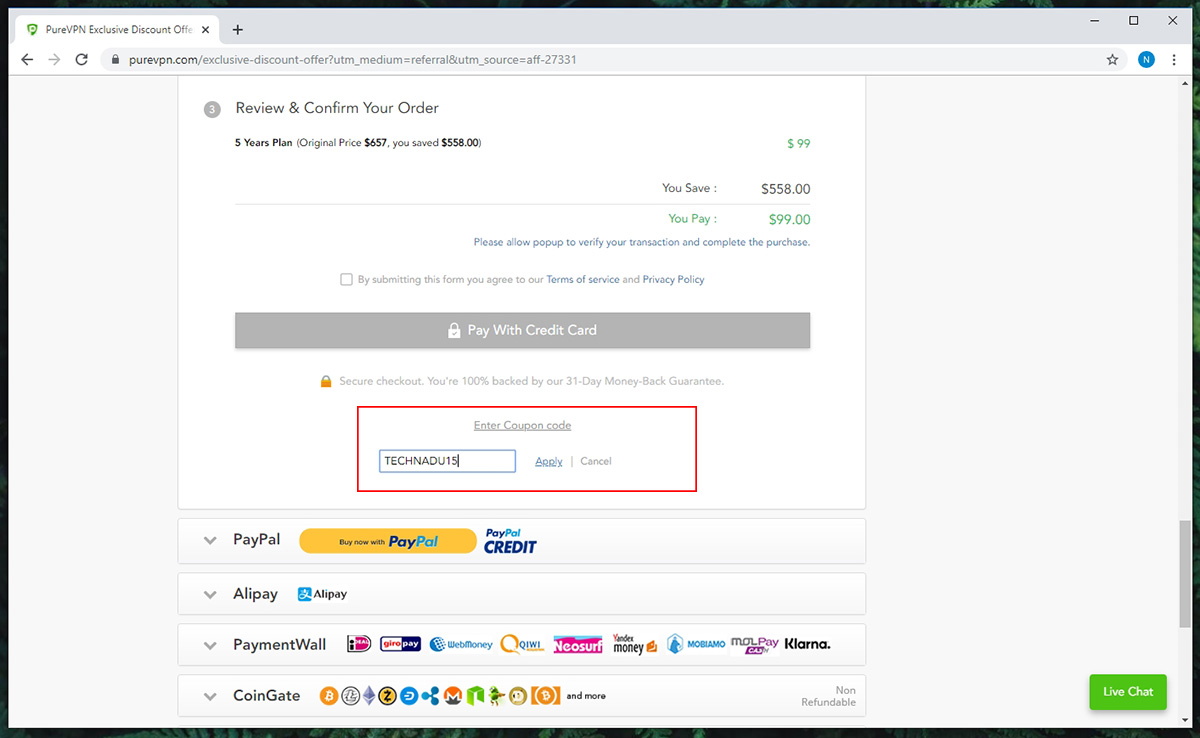The image showcases a payment panel on PureVPN.com's checkout page. The user has scrolled down to the "Review and Confirm Your Order" section, focusing on a five-year subscription plan. The original price of the plan is $657, but an exclusive discount reduces it to $99, offering a substantial saving of $558. Terms and conditions selection options are visible.

A prominent gray button allows for credit card payment. Below this, the "Secure Checkout" notice includes a 31-day money-back guarantee. A highlighted red rectangle surrounds a coupon code field with "TECHNADIU15" entered into it. 

Payment options include PayPal, Alipay, PaymentWall, and CoinGate. Each option is visually distinctive: PayPal features a large yellow button and a PayPal Credit link, Alipay shows its own logo, PaymentWall displays several logos, and CoinGate is accompanied by a row of Bitcoin-related icons. 

In the lower-right corner, there is a light green button for live chat, featuring a drop-down menu. The browser itself has a visible scroll bar on the right side.